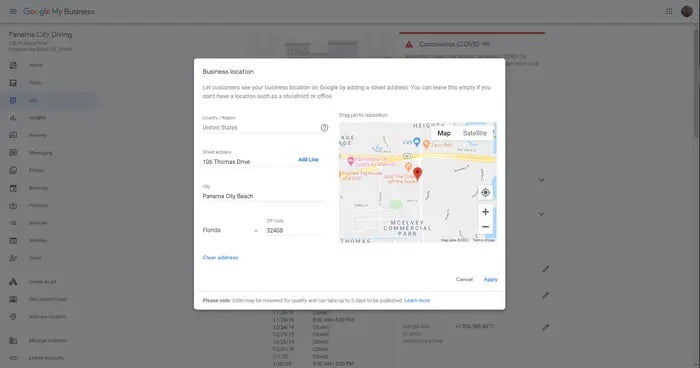The image is a low-resolution screenshot of a Google My Business web page, characterized by a subtle gray filter over the background. In the upper-left corner, the Google My Business logo is prominently displayed. A vertical menu on the left side features various navigation options, with "Panama City Driving" clearly visible among them. Other menu items include icons, such as a calendar icon, and possible text options like "Bookings," though the resolution makes it challenging to discern the details.

On the right side of the screenshot, there is an orange notification bar warning about COVID-19, indicated by an orange triangle with an exclamation mark, followed by the text "Coronavirus (COVID-19)." While there is additional information below this notification, the text is too blurred to read clearly.

In the top-right corner, a circular icon likely represents the user’s profile thumbnail. The center of the image features a bright white rectangular pop-up with text. The header of this pop-up reads "Business Location" and prompts users to "Let customers see your business location on Google by adding a street address." It advises leaving the field empty if there is no physical location like a storefront or office. Below this instruction, the address fields are filled in with "United States," "106 Thomas Drive, Panama City Beach, Florida 32408."